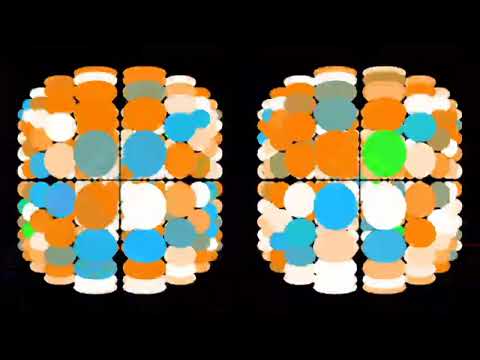The image is a computer-generated digital rendering set against a completely black background, featuring two abstract, square-like objects. Each of these square-like entities is constructed from an intricate collage of hundreds of overlapping circular shapes in various colors, including orange, white, muted blue, muted orange, gray, and neon green. The objects are reminiscent of Rubik's Cubes, segmented into four quadrants by plus sign dividers. Despite their abstract nature, the circles are meticulously layered and stacked, creating a visually complex and artful design. Notably, a single green dot is seen on the square on the right. The absence of text emphasizes the focus on the vivid and diverse color palette, enhancing the image's artistic appeal.